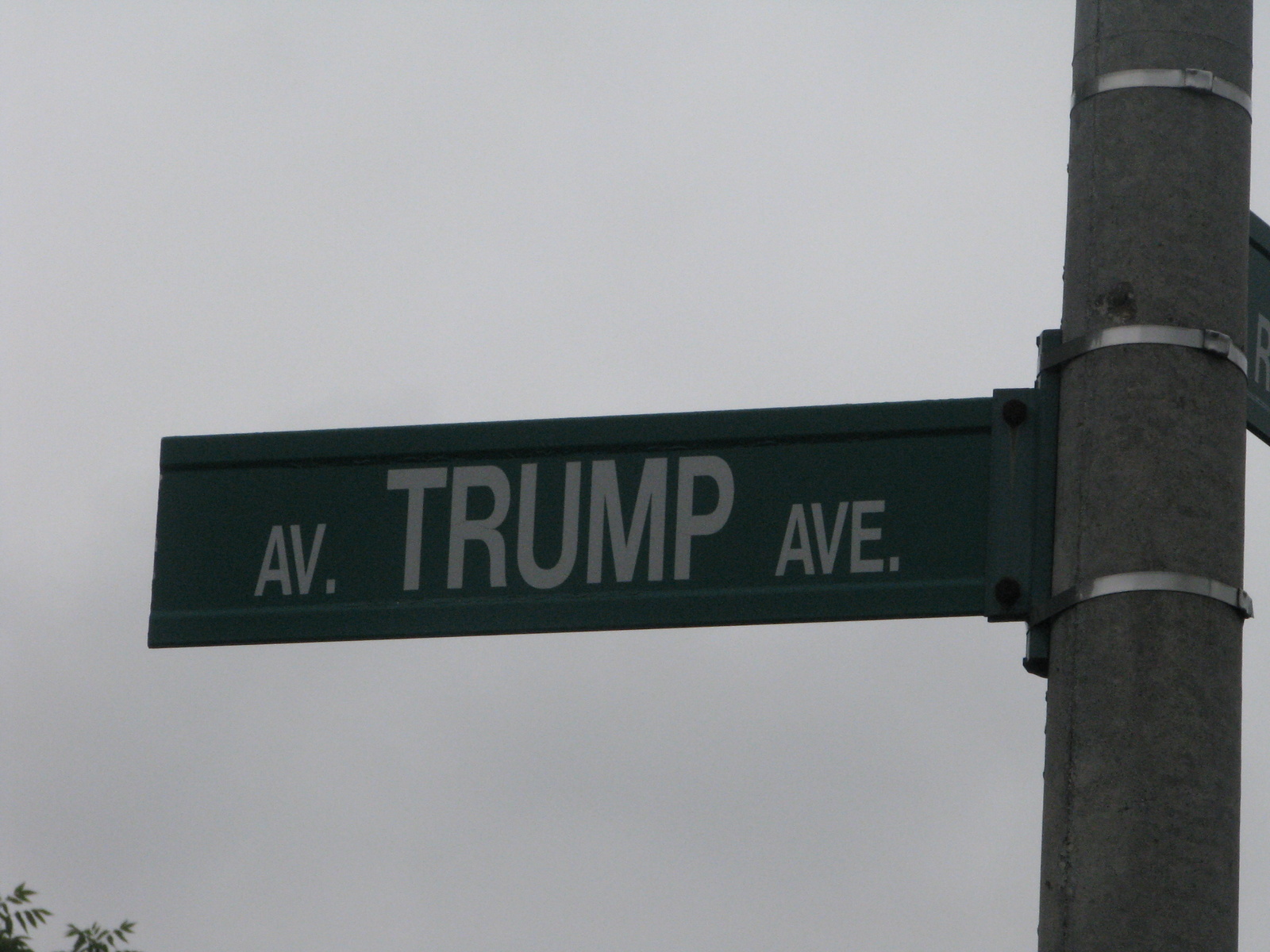The photograph captures a dull, grayish-toned scene dominated by a green street sign that reads "Trump Ave." The sign is a long, thin rectangle with the "Ave" followed by a dot. In the bottom left corner of the image, small branches with leaves provide a natural contrast to the otherwise muted colors. The sign is mounted on a sturdy pole, possibly made of metal or concrete, secured by three metal ties. While the two ties firmly hold the Trump Ave sign, the third tie hints at another sign on the opposite side of the pole. However, only an indistinct partial letter, possibly a P or R, is visible from this angle.